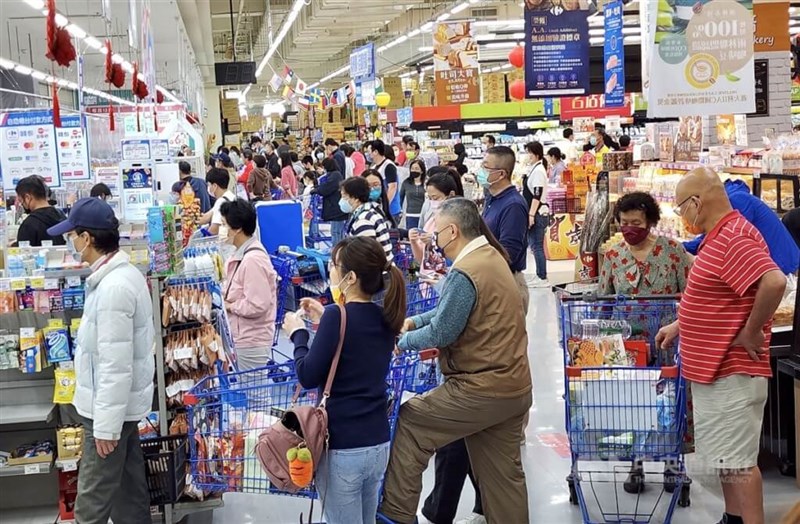The image depicts a bustling, warehouse-style supermarket, likely located in either China or Japan, indicated by the Asian lettering on hanging signage and the predominantly Asian shoppers, many of whom appear to be middle-aged or older. The spacious, high-ceilinged interior is filled with numerous products and thick with the presence of blue shopping carts laden with groceries. The crowd is significant; all checkout registers are open, with about five masked individuals waiting in each line – a testament to the pandemic era when the photo was taken. In the foreground, a man in a white jacket and blue baseball cap leads one queue, followed by a woman in a dark blue sweater and ponytail, and then a couple, the man wearing a brown vest over a blue shirt. The atmosphere is animated and tightly packed, evoking a sense of organized chaos as everyone moves toward the checkout lines to complete their purchases.